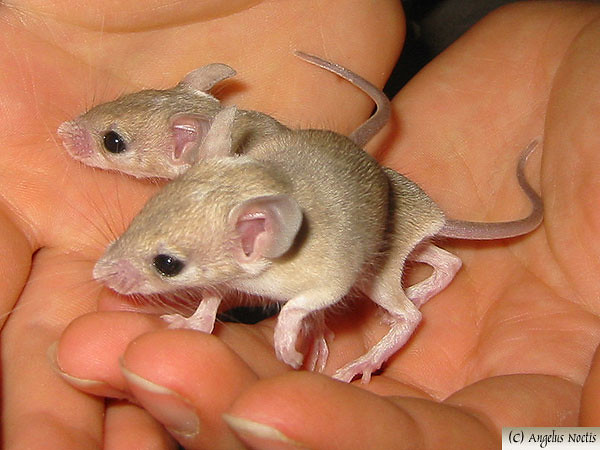In this very detailed close-up image, two hands are clasped together, palms up, gently cradling two small mice. The hands are cupped, with one resting on top of the other to create a cozy space for the tiny animals. The mice appear to be babies, featuring large ears and tiny pink feet. Their bodies are primarily gray with white underbellies, and they have short, barely formed tails. The mice have wispy, spiky hair and long whiskers, adding to their delicate appearance. Both appear content and are nestled closely together, with one mouse partially obscuring the other. In the lower right corner of the image, there is a white rectangular box containing a C copyright symbol and the name "Angelus Nostris" in black writing.